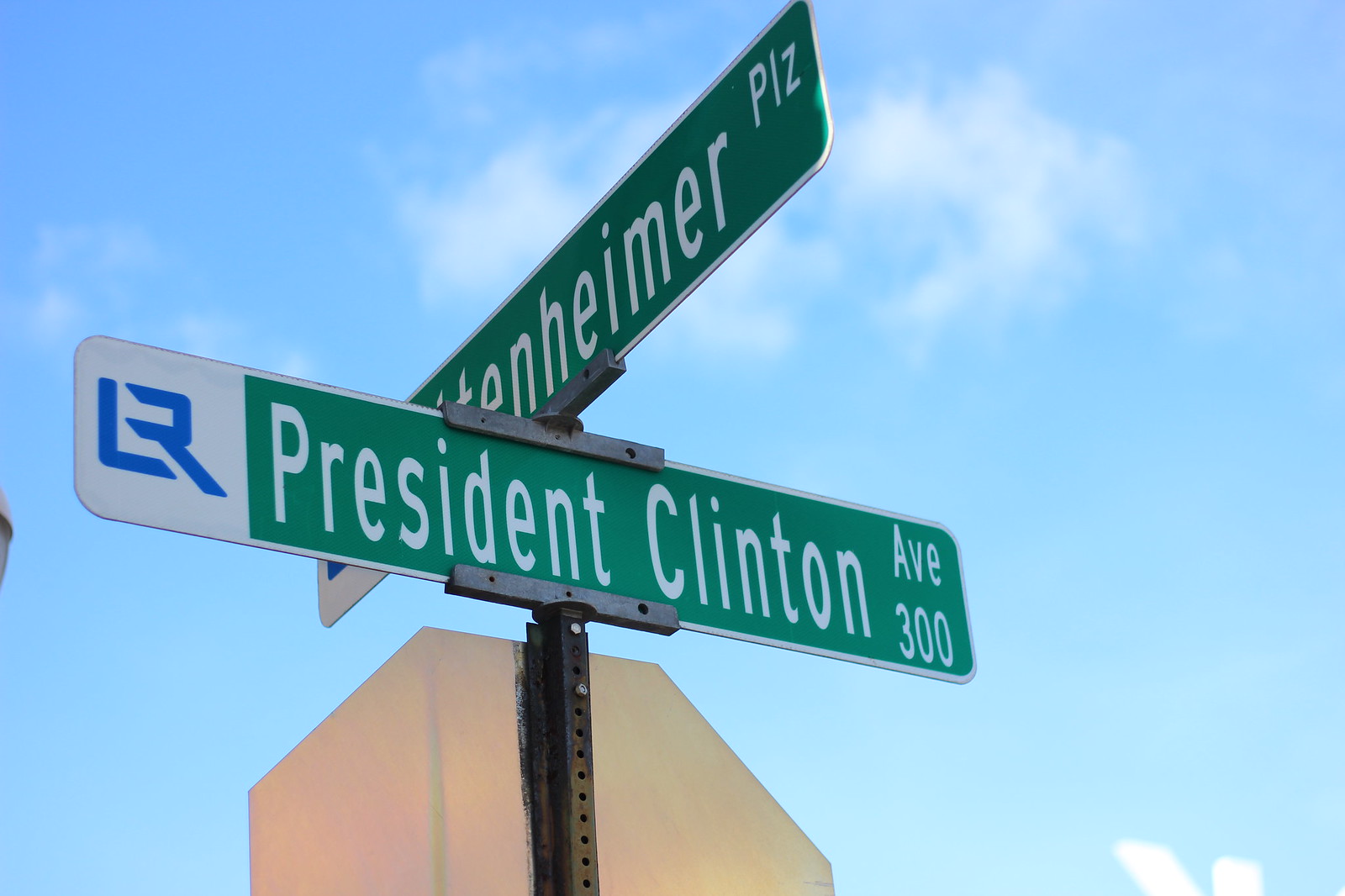A serene daytime scene showcases two intersecting street signs set against a vibrant blue sky punctuated with a few gentle clouds. The primary focus is on the two rectangular, green street signs mounted perpendicularly. The upper sign, slightly difficult to decipher, reads "TENHEIMER PLZ" in white lettering. Below it, the clearly legible sign reads "President Clinton Ave 300" in bold white letters. On the left side of the lower sign, a blue emblem features an intricate design resembling the combination of an L and an R. The signs are affixed to a dark green or black signpost, replete with visible holes for mounting screws, which adds to the functional charm of the urban landscape. In the background, we catch a glimpse of the back of a stop sign, its unmistakable octagonal shape suggested by the visible white border. This street corner combines both the everyday simplicity and the subtle details of city life on a pleasant day.